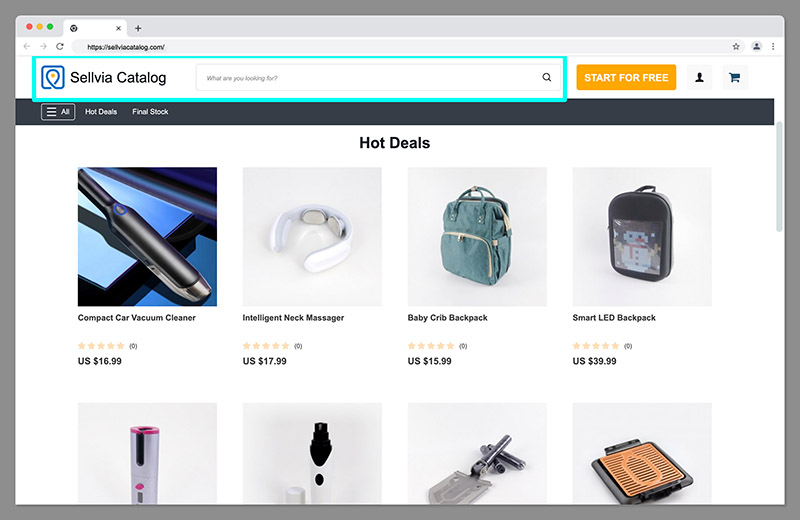On the website https://selviacatalog.com, the homepage features a neatly organized layout. Beneath the prominent URL 'https://selviacatalog.com,' spelled out as S-E-L-L-V-I-A, is a user-annotated blue-turquoise box bearing the distinctive Selvia logo. The logo consists of a square encapsulating an upside-down teardrop symbol, akin to a location icon, highlighted by a yellow star at its center.

Centered on the page lies a search bar with the placeholder text "What are you looking for?" in light gray italics. Adjacent to the search bar, there's a gold button labeled "Start for Free." Following this, a small square button featuring a user icon is present, and next to it is a blue shopping cart icon.

Above these elements, a sleek, black-colored menu bar with white text includes a hamburger icon and options labeled "All," "Hot Deals," and "Final Stock." Displayed predominantly across the midsection of the webpage are various current hot deals. There are a total of eight product icons, though only the top four are fully visible. These products include:

1. A compact car vacuum cleaner priced at $16.99, though no user reviews are available.
2. A neck massager positioned to the right of the vacuum cleaner.
3. A baby crib backpack next to the neck massager.
4. A smart LED backpack priced at $39.99 on the far right.

The webpage is designed to showcase these deals attractively, likely to capture the user's attention and encourage exploration of the website's offerings.